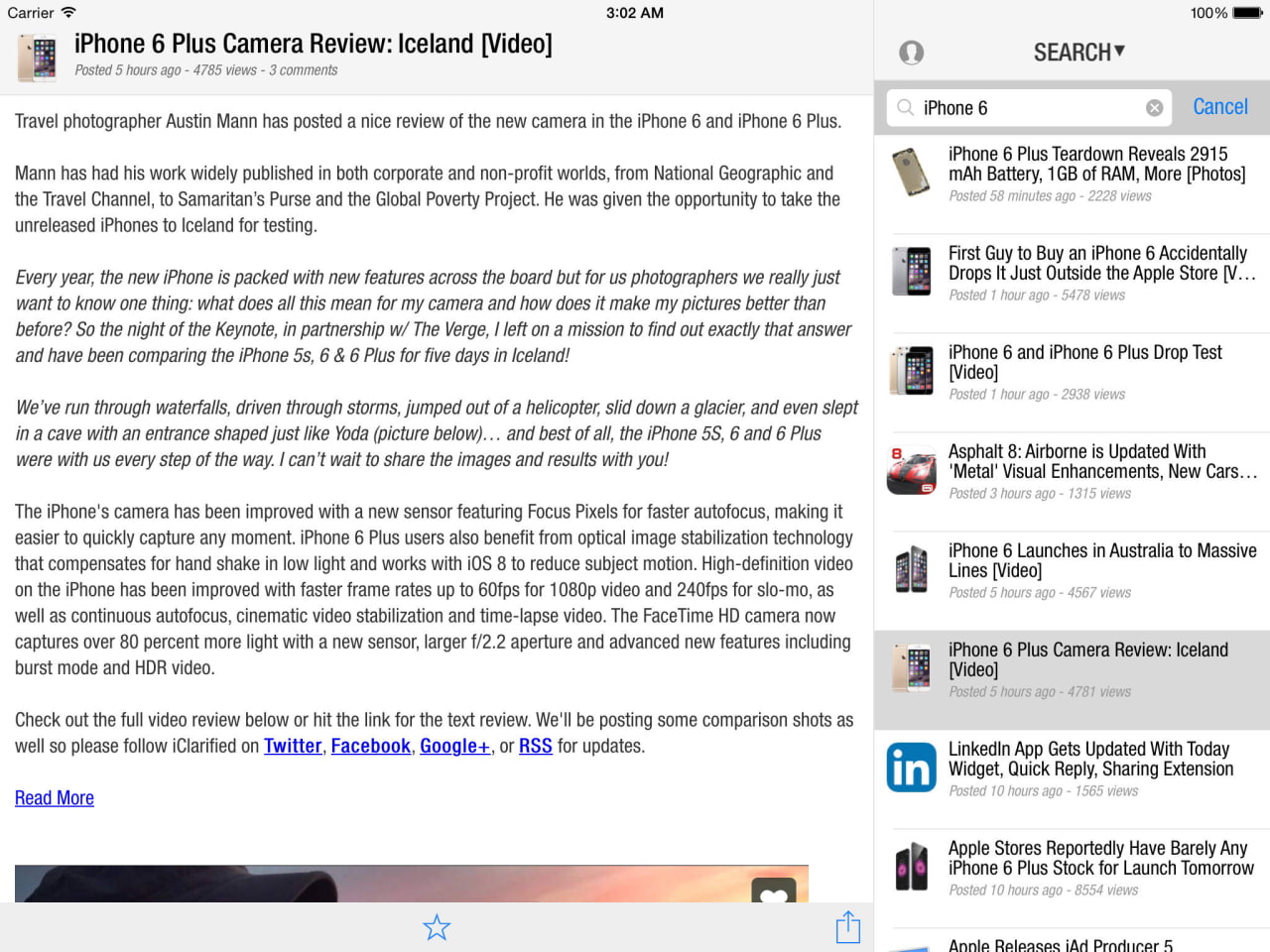Travel photographer Austin Mann has posted an in-depth review of the iPhone 6 and iPhone 6 Plus cameras, showcasing their capabilities during his trip to Iceland. The video, which was uploaded 5 hours ago and has already garnered 1,795 views and 3 comments, highlights the camera's performance in various challenging conditions.

Mann, participating in the Travel Challenge, extensively tested the iPhone 6 Plus camera, which boasts improved features such as a new sensor with focus pixels for faster autofocus and optical image stabilization technology for better photo quality. He compared the iPhone 5 and iPhone 6 over a series of rigorous tests, including photographing through storms and from helicopters, emphasizing that the new camera's agile optimization significantly enhances picture quality.

With a fully charged battery and reliable Wi-Fi connectivity through 2 AM, Mann documented his experiences, noting how the camera's advancements make capturing moments more seamless. His review is a valuable resource for both corporate and non-corporate applications, as he illustrates the practical benefits of the upgraded camera technology.

For more detailed insights, watch the full video where Mann discusses how the enhanced features of the iPhone 6 Plus have improved his photography, and explains why it’s a worthy upgrade for travel photographers and enthusiasts alike.